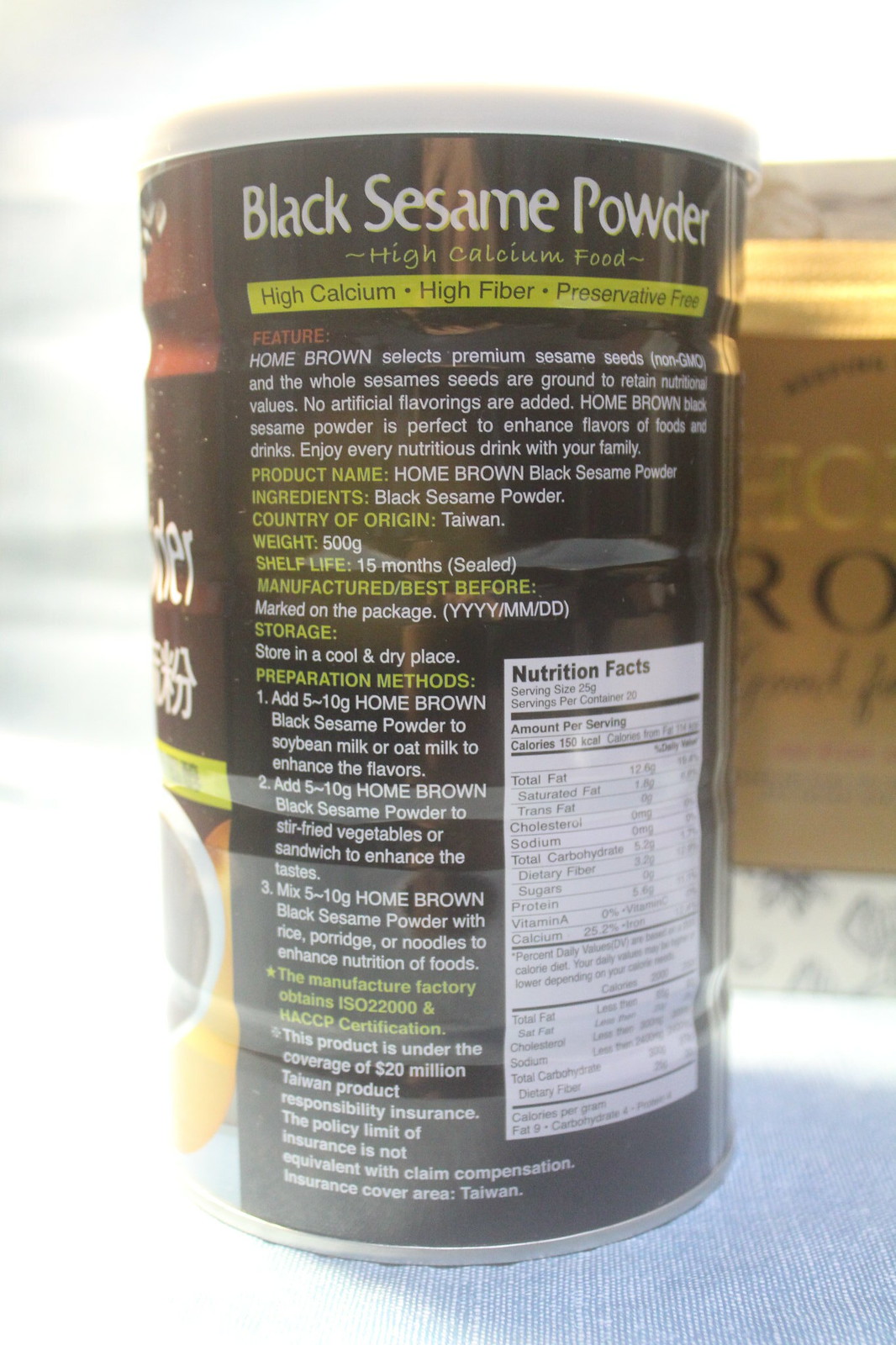The photograph features a sleek, cylindrical container of black sesame powder, made from metal with a contrasting white plastic top. The container itself is a deep black, adorned with a matching black label. Bold white typography prominently announces "Black Sesame Powder" at the top of the label. Underneath this, also in white, the label highlights that the product is a "High Calcium Food." A light green strip beneath these declarations carries additional benefits in black text, listing the product as "High Calcium, High Fiber, and Preservative Free."

Further descriptive information about the black sesame powder, including product name, shelf life, storage instructions, and preparation methods, is presented in a combination of lighter green and white fonts. To the right on the label, a white rectangular section houses the nutritional facts in black text, detailing elements like total fat, cholesterol, sodium, as well as the vitamins and minerals contained within the product.

The container is placed on a blue tablecloth, providing a contrasting backdrop that enhances the product's visibility. In the background, a gold kitchen sign adds a touch of warmth and homeliness to the setting.